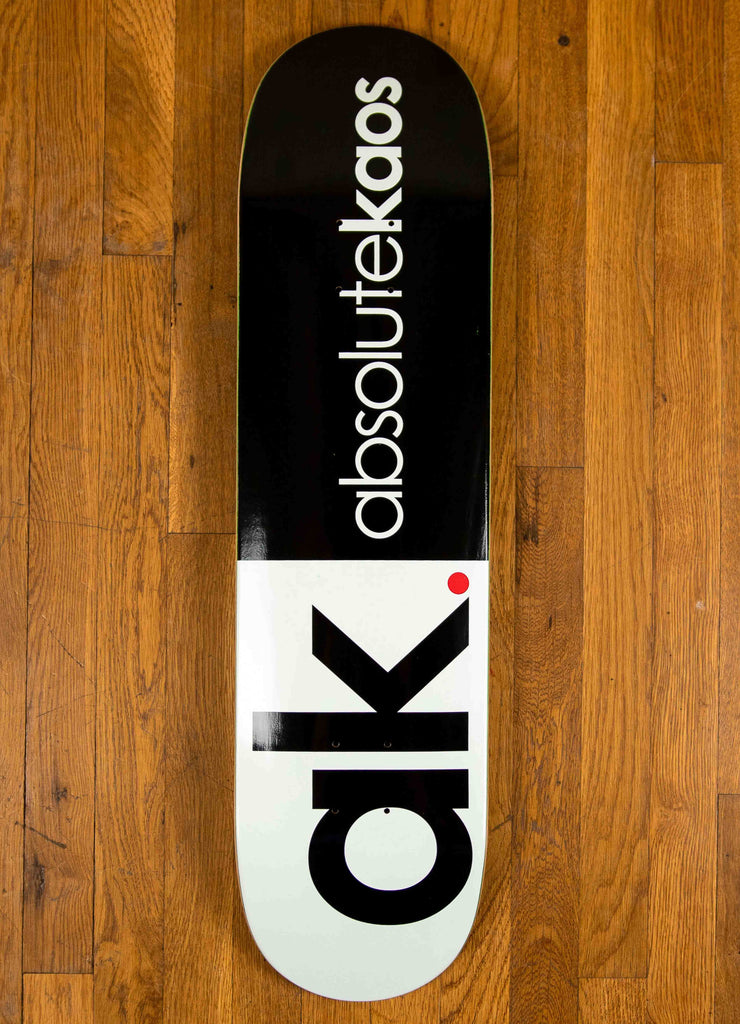The photograph captures a skateboard placed on a wooden floor composed of rectangular planks in varying shades of brown, revealing distinct wood grain patterns and some black spots. The skateboard's deck is divided into two sections: the lower third features a white background with the black lowercase letters "ak" followed by a red period, while the upper two-thirds displays a black background with the phrase "Absolute Chaos" in smaller, white, uppercase letters, with "Chaos" spelled as "K-A-O-S." The image appears to be taken in a home setting, as suggested by the light reflecting on the skateboard's white section.